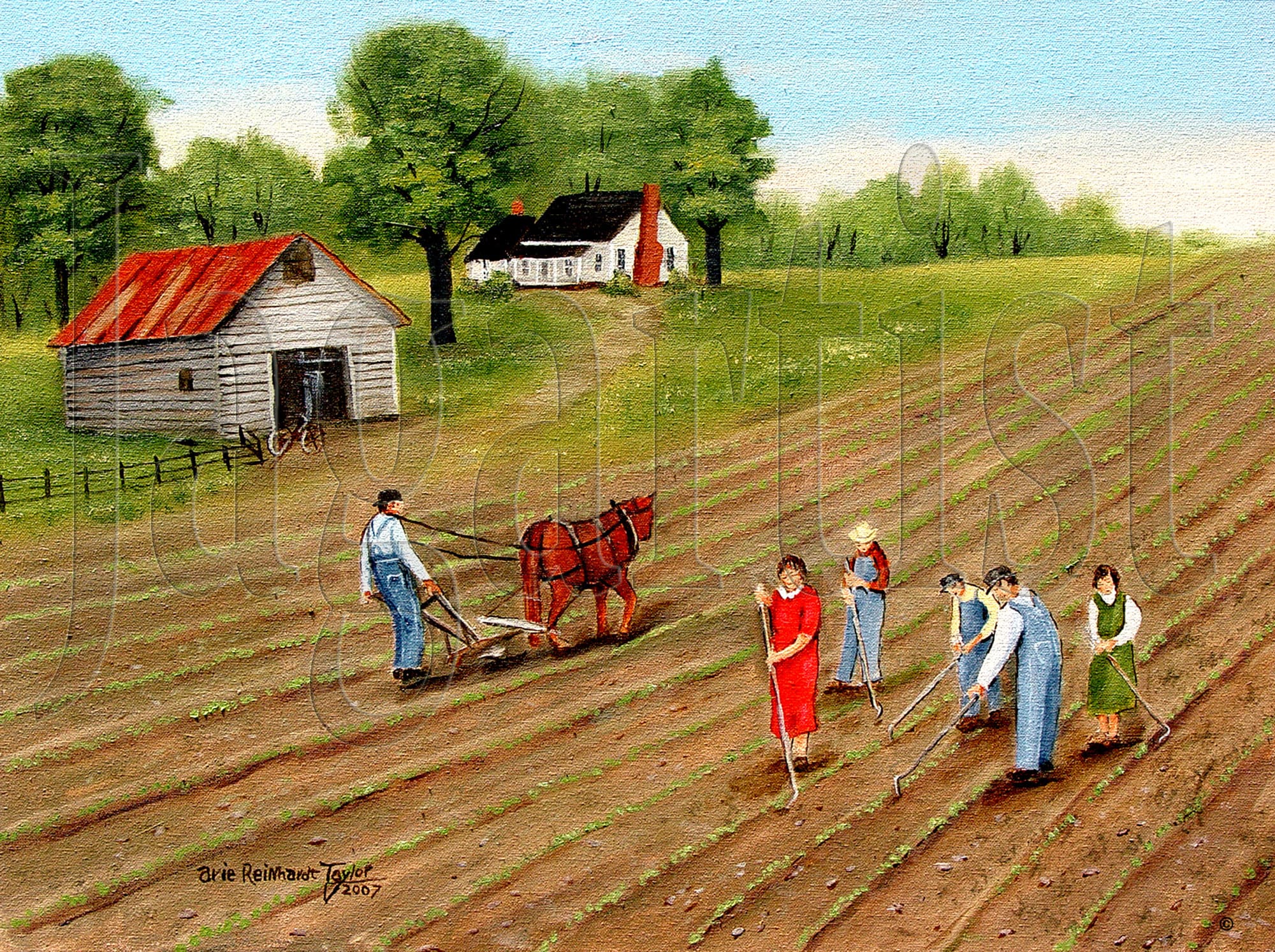This is a richly detailed, horizontal color painting depicting a bustling farmland scene. In the foreground, five people are seen diligently plowing the land with hand hoes; they are dressed in a mix of red dresses, green dresses, and jean overalls. To their left, a man in jean overalls and a black hat leads a brown horse pulling a plow. The farmland is adorned with horizontal rows of lush green crops that stretch towards the horizon.

On the left side of the painting stands a white wooden barn with a distinctive red metal roof and a prominent central door, flanked by a black fence. A bicycle leans against the barn, adding a touch of rustic charm. Behind the barn, various green trees provide a verdant backdrop.

Further back, nestled among these trees, is a quaint white house characterized by its black roof and red brick chimney. This cottage-style house features numerous windows and exudes a serene, pastoral elegance. Above, the sky is a pretty blue, completing this idyllic depiction of rural life.